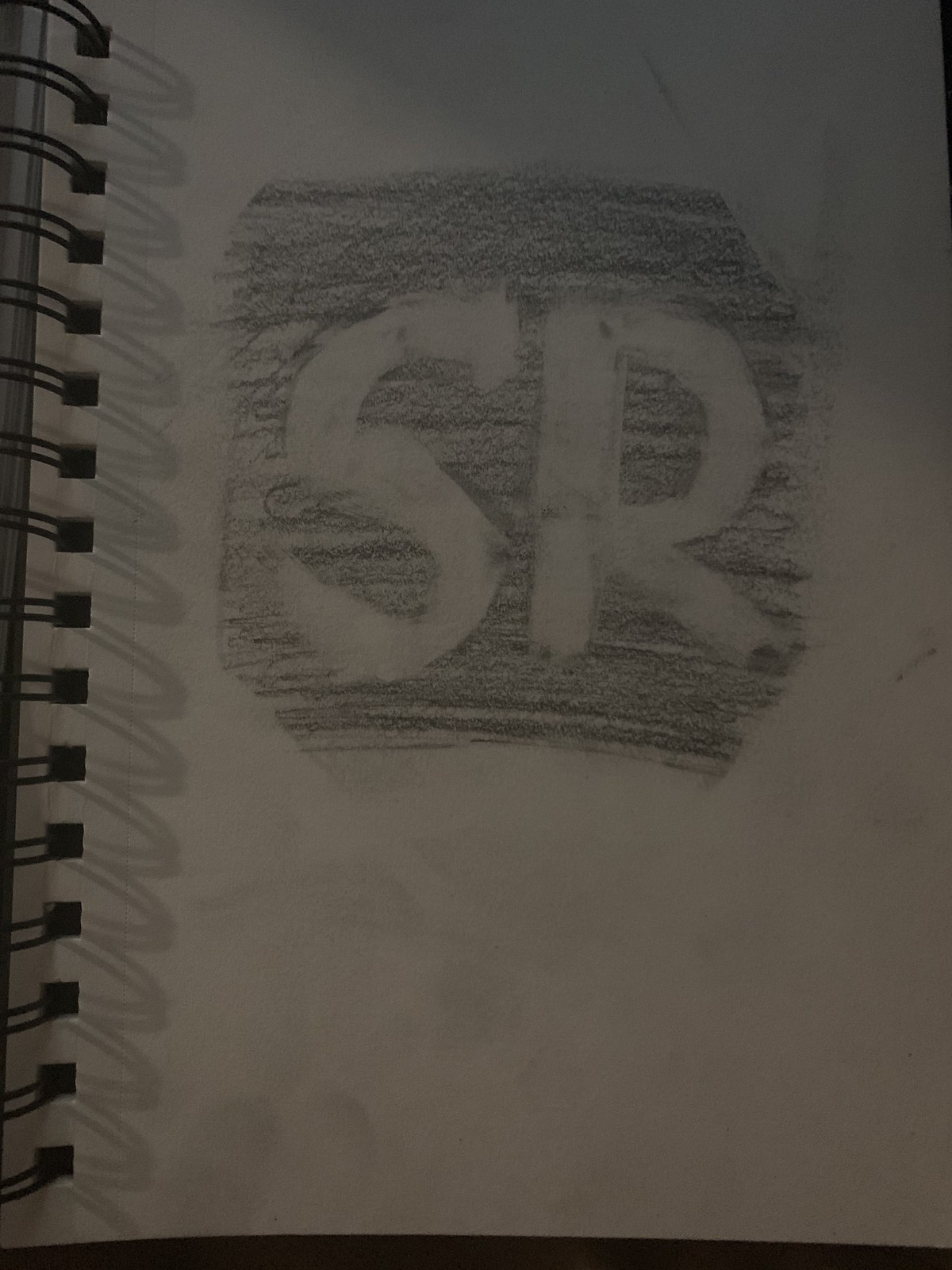In this image, we observe a large, intricate scribble drawn on a blank, white notebook page. The notebook features a spiral spine on the left-hand side. The scribble forms a hexagonal shape, created with a graphite pencil. At the center of the hexagon, the artist has meticulously erased a portion to reveal the letters "S" and "R." The positioning and depth of the shadows indicate that the primary light source is situated to the left of the photographer.